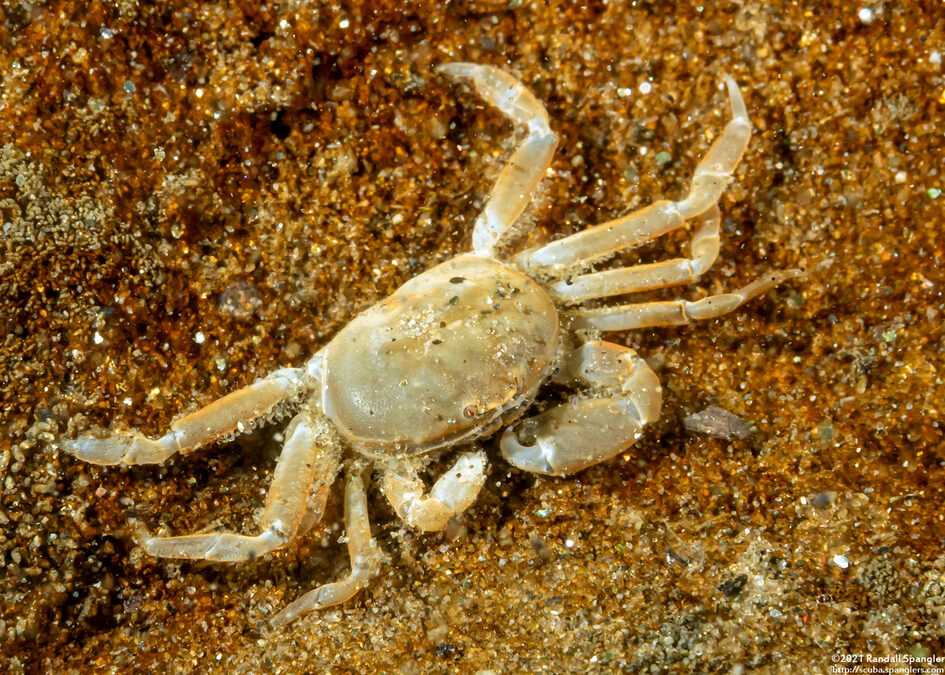The photograph is a close-up, rectangular image featuring a small, semi-transparent crab in the center. The crab, largely tan with some white ridges and sections, blends seamlessly with its surroundings—a fine mix of brown, black, and tan sand grains. It has a stick-shaped body with four legs on either side and two arms at the front; one arm has a large curved pincer, while the other is smaller and more maneuverable. The sandy surface around the crab appears brownish-orange, giving the impression of a beach or rock formation. Though the crab appears still and its eyes are not visible, the intricate details of its translucent body and the fine grains of sand provide a rich texture to the image. In the bottom right corner, there is small white text, too small to be legible.